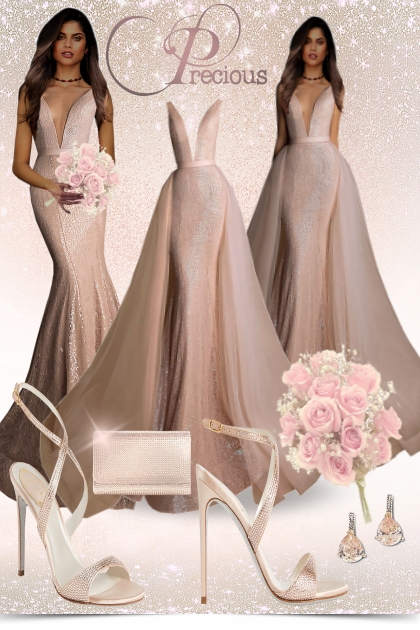The image titled "Precious" is an intricately designed advertisement featuring an elaborate evening or wedding gown alongside matching accessories. The background is a pink and white sparkly gradient adorned with glittery stars, creating a glamorous ambiance. The word "Precious" is elegantly displayed at the top center, with its ornate "P" emitting intricate lines that frame the scene.

In the visual, there are two depictions of the same woman wearing the luxurious gown. On the left, she holds a bouquet of light pink flowers, showcasing the form-fitting, strapless dress with a plunging V-neckline that accentuates her waist before flaring out into a bell shape at the knees. The gown is a glittery beige fabric that sparkles under the light. 

On the right, the same woman appears with her hands behind her, and the dress is shown with an additional lighter material attached to the waist, giving it a fuller appearance. Her long brown hair cascades elegantly down her back in both instances.

Central to the image is a standalone view of the dress on a mannequin, emphasizing its design and intricate details. Surrounding this centerpiece are matching beige high-heeled sandals, a white clutch purse with a subtle shimmer from the top left corner, and a pair of pink blush teardrop earrings positioned near the flowers on the right. This detailed layout highlights the harmonious blend of elegance and glamour, ensuring the viewer's focus on the complete ensemble.